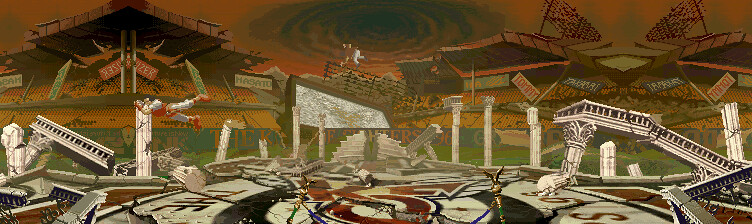The image depicts a devastated, panoramic scene reminiscent of a post-apocalyptic arena, likely a reference to a stage from the King of Fighters game series. Dominated by deep rust red and dark green hues, the sky features a swirling vortex, resembling a tornado or hurricane. Beneath this ominous atmosphere lies the crumbling remains of a city, with architecture inspired by ancient Greek designs. The cityscape is filled with dilapidated marble or white-stone buildings, cracked and fallen pillars, and crumbled statues.

Amidst the destruction is a once-majestic colosseum, now in ruins. The center of the colosseum is marked by a circular formation ascending into the sky, strewn with debris. Visible on one of the broken columns is a figure clinging desperately, wearing an orange shirt over a gray shirt, gray pants, and orange shoes. The far background reveals fractured seating areas, collapsed sections of the ceiling, and additional cracks scattered across the desolate ground. In the top-center of the sky, a black hole-like feature adds to the scene's apocalyptic ambiance, with another figure being drawn towards it, clad in a brown shirt and white pants. This richly detailed image captures the essence of a world torn apart, equal parts haunting and mesmerizing.